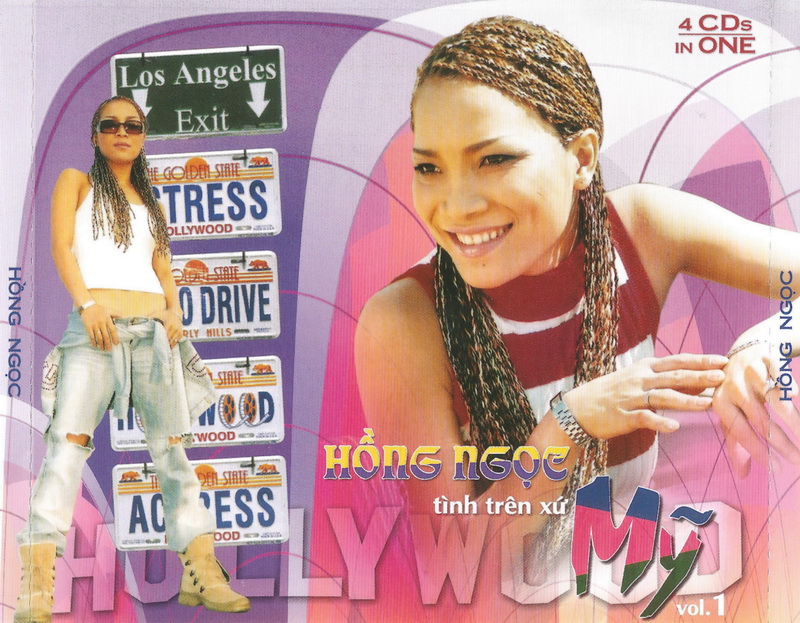The image depicts a CD cover showcasing a light-skinned African-American woman with cornrow hair extending past her ears and down to her chest. The cover is divided into two sections: the left section features her standing with feet spread in beige ankle boots, light blue jeans torn at the knees, and a white sleeveless tank top, accessorized with a bracelet on her right wrist and dark brown sunglasses. The background shows a street sign reading "Los Angeles" and "Exit," alongside various license plate-like images, some of which are partially obscured.

The right section presents a close-up of the same woman, highlighting her bare shoulders and a maroon tank top with white horizontal stripes. She also appears to be wearing a watch. The top right corner of the cover states "4 CDs" in red letters against a white background. Her name, "Hang Ngoc," appears prominently on the cover, with a Vietnamese name "Trinh Tin Trinh Xu" written in white letters underneath. The very bottom of the cover displays the word "Hollywood" lightly imposed in white letters across the design. The background is a vibrant mix of purple, blue, and pink patterns.